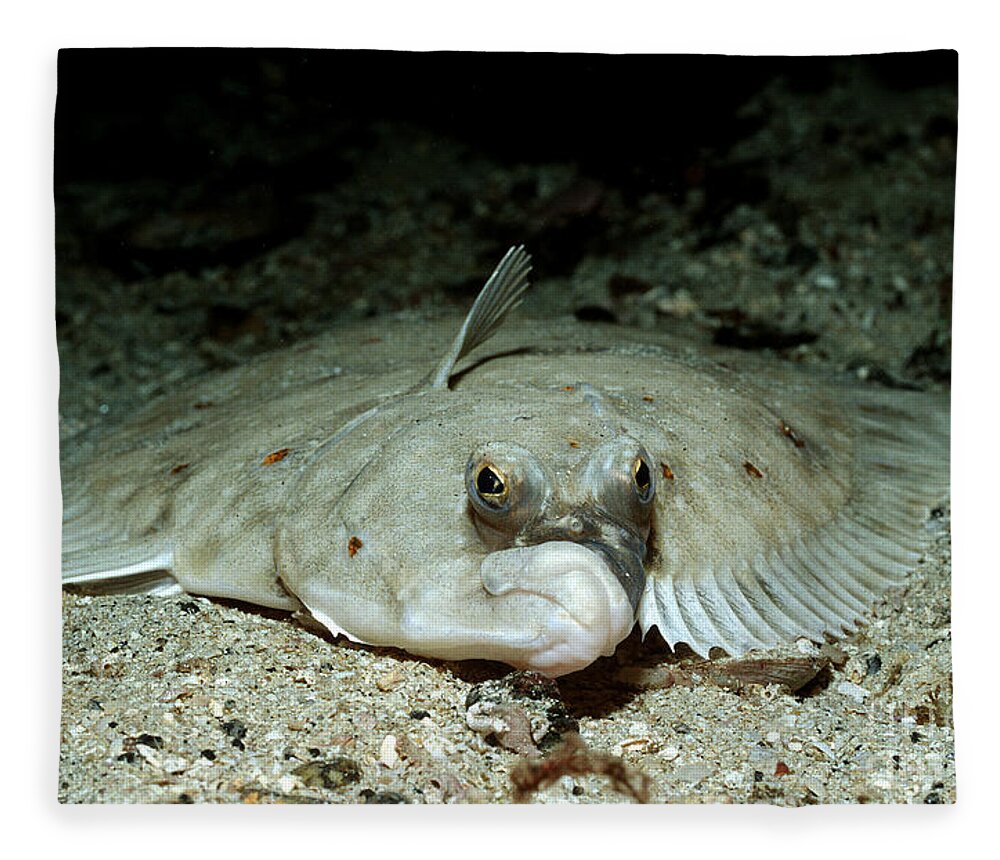This full-color underwater photograph, taken from the ocean floor using artificial light, captures a flat, weird light-brown fish blending seamlessly into a rough and gritty sandy seabed scattered with pebbles, rocks, and broken shells. The square image features wavy borders, enhancing its unique aesthetic. The upper portion of the photo is shrouded in darkness due to the depth and lack of natural light. The fish, with a cream-colored body adorned with fewer than ten small brown spots, lies flat against the seabed like a pancake. It has golden eyes with black pupils and a black nose area. Its body, large and flat, is edged with ribbon-like, ruffled fins. The perspective of the shot is front-facing, allowing a clear view of the fish's details and its harmonious blending with the sandy environment.